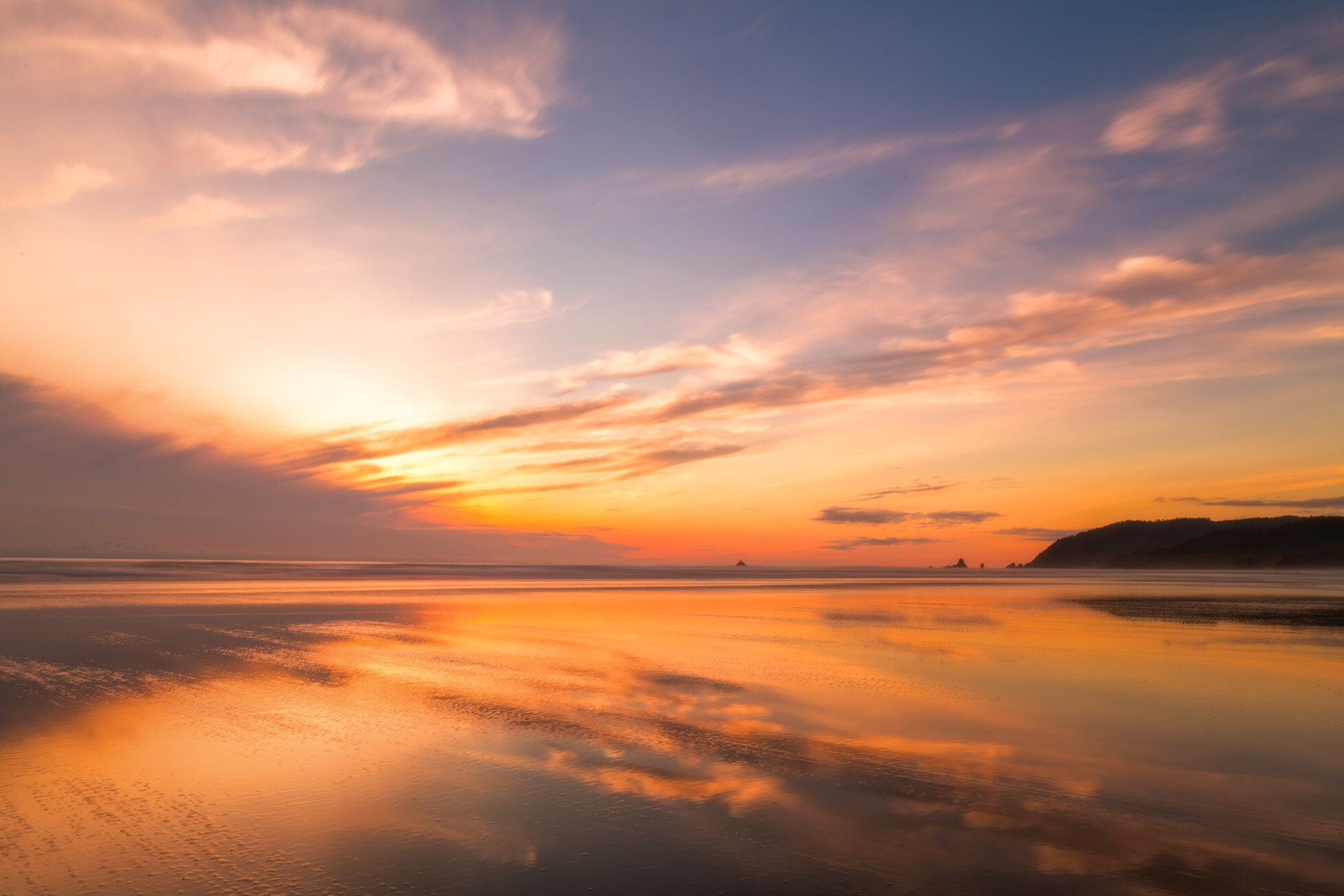This image captures a stunning sunset over a tranquil beach or large lake. The sky is a rich blend of blues, oranges, and yellows, with fluffy clouds scattered throughout, some of which obscure the sun as it sets. The sun's deep orange glow transitions smoothly into shades of yellow and white, creating a mesmerizing gradient. Reflections of this vibrant sky dance on the still, shallow waters that flood the beach, enhancing the serene atmosphere.

To the left, towards the top, the sky remains predominantly blue. On the horizon, a mountain or cliff-like structure dominates the middle of the image, partially blocking the sky and sun. Further right, another hill or rocky coastline juts out into the water, adding depth to the scene. In the far distance, a few silhouettes of ships can be faintly discerned, adding an element of intrigue.

Overall, the image is a harmonious blend of natural elements—water, sky, and land—bathed in the warm hues of a setting sun, all captured on what appears to be a partly cloudy evening.